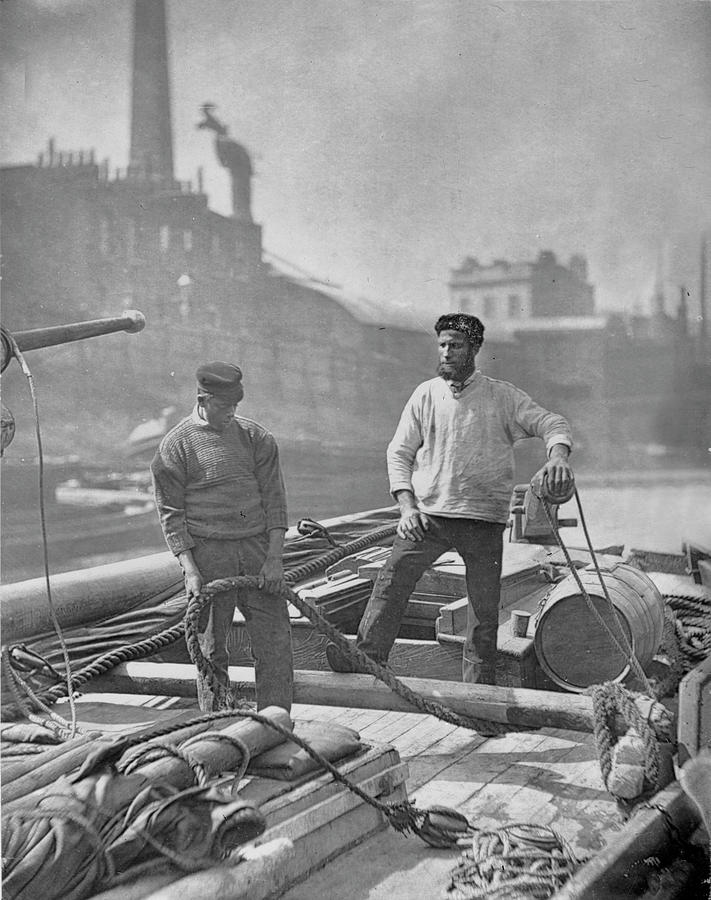This black and white photograph, likely taken during the industrial era, features two sailors working on a barge in an industrial harbor. One man, dressed in a dark cap, sweater, and pants, is coiling a thick rope, while the other, wearing a beanie and a white sweater, steadies himself with his leg on a post and grasps a handle that seems to be part of a steering mechanism. The deck is cluttered with barrels and sails lying down, and numerous ropes are visible, likely used to secure the mast and connect to the pier. In the background, large factories with smoke billowing from their smokestacks dominate the shoreline, contributing to the smoky, industrial atmosphere.